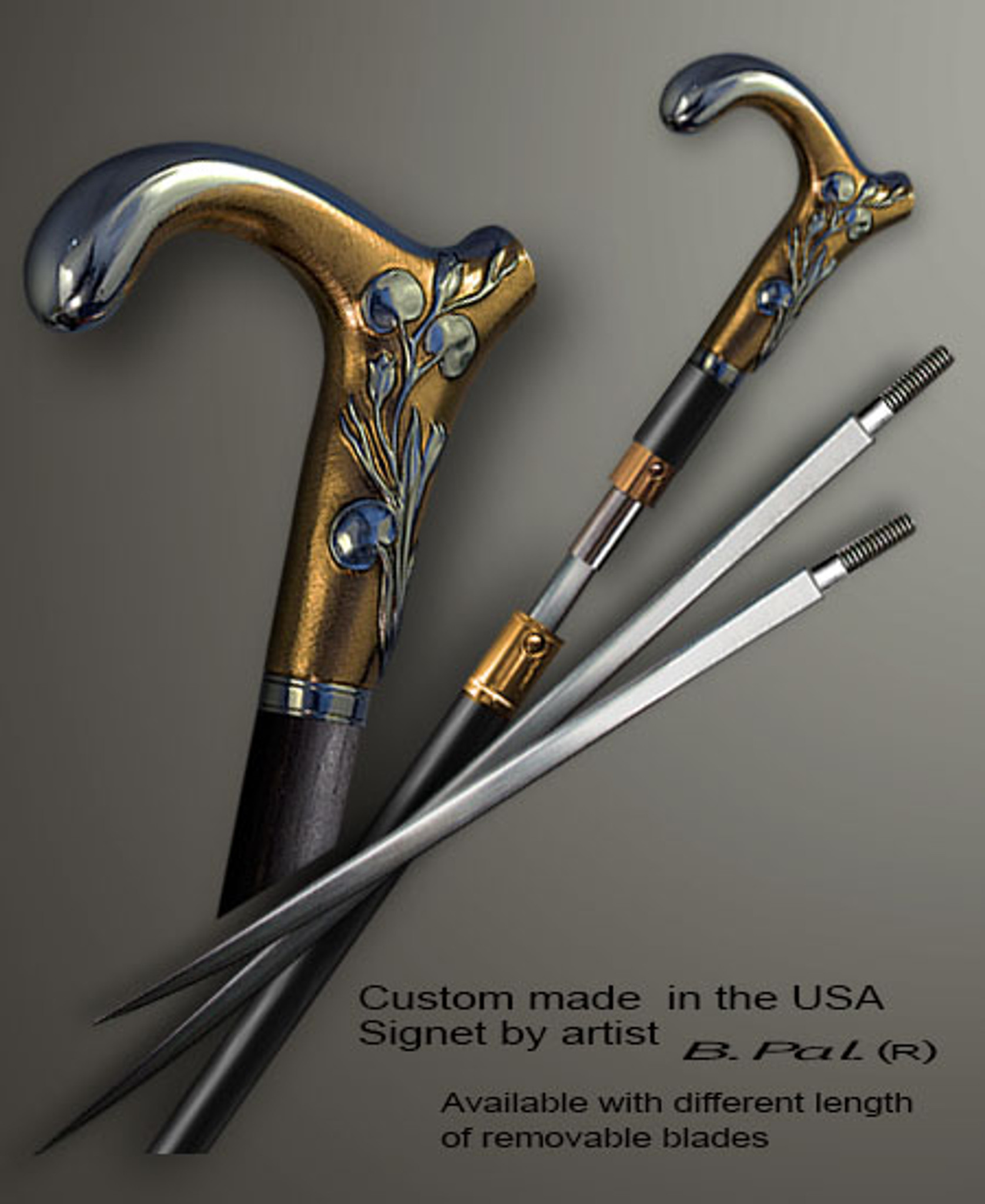This photograph, which serves as an advertisement, features a collection of custom-made, artisan blades and their accompanying handle crafted in the USA by artist B Powell. Dominating the image is an ornate, cane-like handle with a circular grip, finished in gold and silver hues. Adorned with intricate engravings resembling flowers or vines accented in bluish colors, the handle presents a luxurious and elegant design. The body of the handle features a dark wood finish complemented by a silver rim. Alongside the handle are three sleek, removable blades, designed to screw into the handle, allowing for customizable lengths. The text on the photo emphasizes the custom craftsmanship and availability of different blade lengths, enhancing the artistic and functional appeal of these specialized tools.